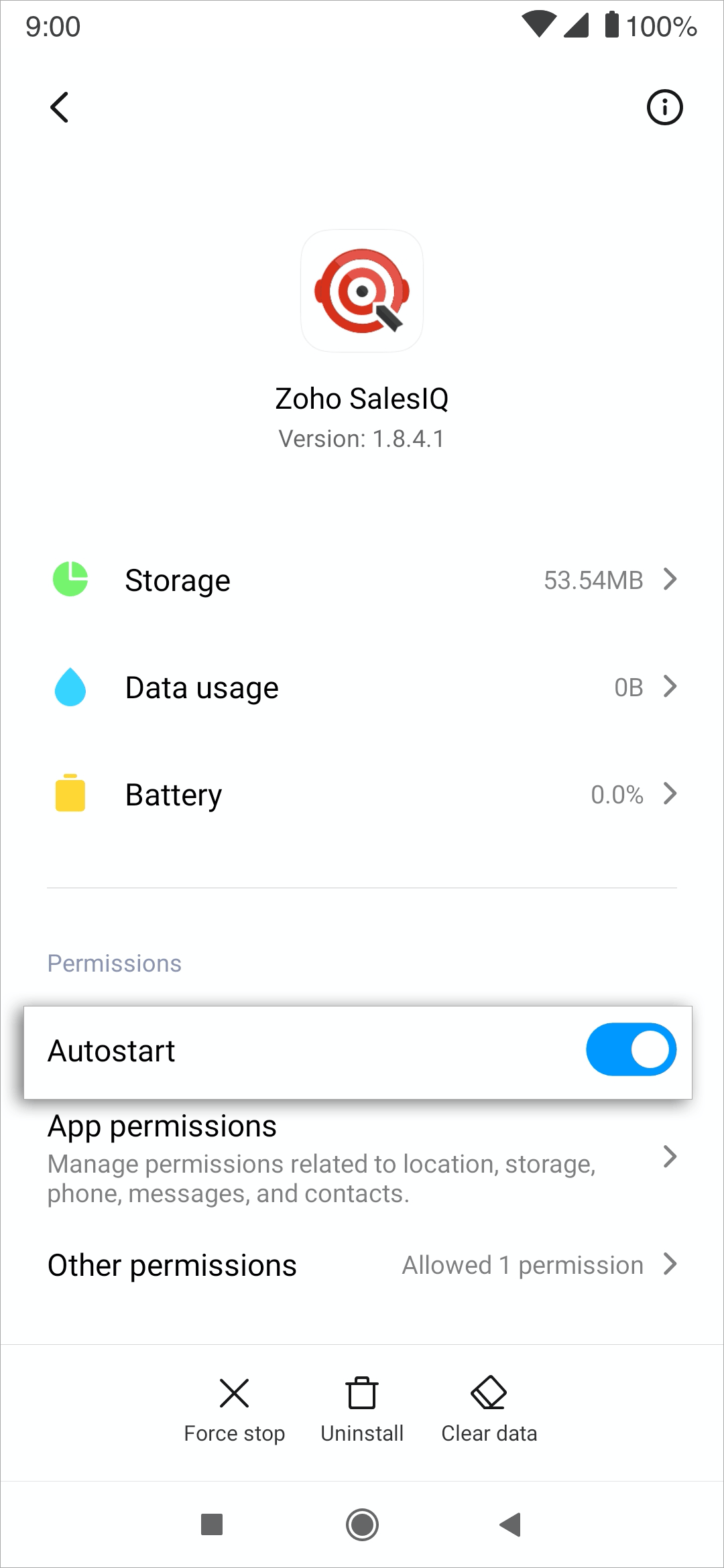A screenshot from a smartphone app, displaying various details and settings for the app "Zoho Cells IQ" (version 1.8.4.1). At the top left corner, the time, battery percentage, and several other icons are visible, indicating the phone's status. The app background is white with a prominent red circular shape at the center, featuring a black dot in the middle.

Beneath the app name and version, several sections are outlined:

1. **Storage Usage**:
   - Displays the app's storage consumption, listing it as 53.54 megabytes.

2. **Data Usage**:
   - Indicates that the app has used 0 bytes of data, accompanied by a small blue icon resembling a water droplet.

3. **Battery Usage**:
   - Shows 0.0% battery usage with a yellow icon.

4. **Permissions**:
   - Contains an auto-start option, marked by a blue box to indicate it is enabled.
   - Offers the ability to manage various app permissions such as location, storage, phone, messages, and contacts.
   - Highlights another permissions section, noting that one permission has been allowed.

5. **App Management**:
   - Includes options for Force Stop (marked by an X), Uninstall (accompanied by a garbage can icon), and Clear Data (illustrated with an eraser icon).

This screenshot provides a comprehensive overview of the app's key statistics and settings, allowing for efficient management and monitoring of its functions on the smartphone.